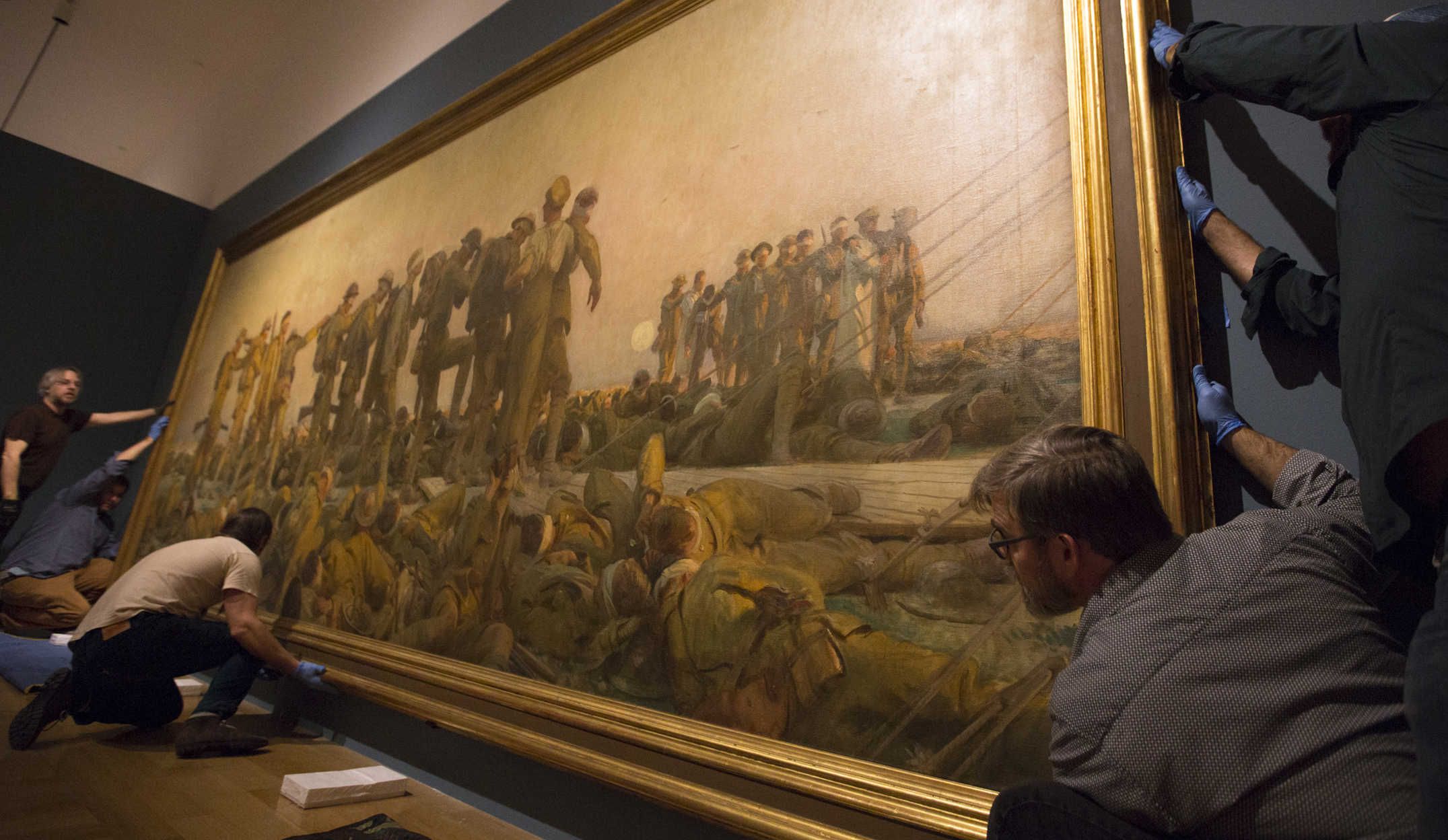The photograph captures a detailed scene in a museum where five men are diligently mounting a large, somber wartime painting on a dark navy blue wall. The perspective is from floor level, revealing a stark white ceiling and light tan wood plank flooring beneath the activity. Each man, dressed in semi-casual business attire, including a man in a blue polka-dotted shirt and another in a tan t-shirt, carefully handles the massive artwork with blue vinyl gloves. The painting, depicting a military scene, is filled with somber imagery: groups of fallen soldiers in green uniforms lie at the bottom, while others, some wounded with head wraps and bandages, stand mournfully above them. The color palette of the painting is muted with ochres, military greens, beiges, and grays, enhancing its somber tone. The men appear to be positioning the painting, possibly preparing to set it down, with additional equipment on the floor hinting at restoration or cleaning efforts. Disembodied hands and partial figures add to the intricate activity captured in the image, reflecting the careful and respectful handling of this significant piece of art.